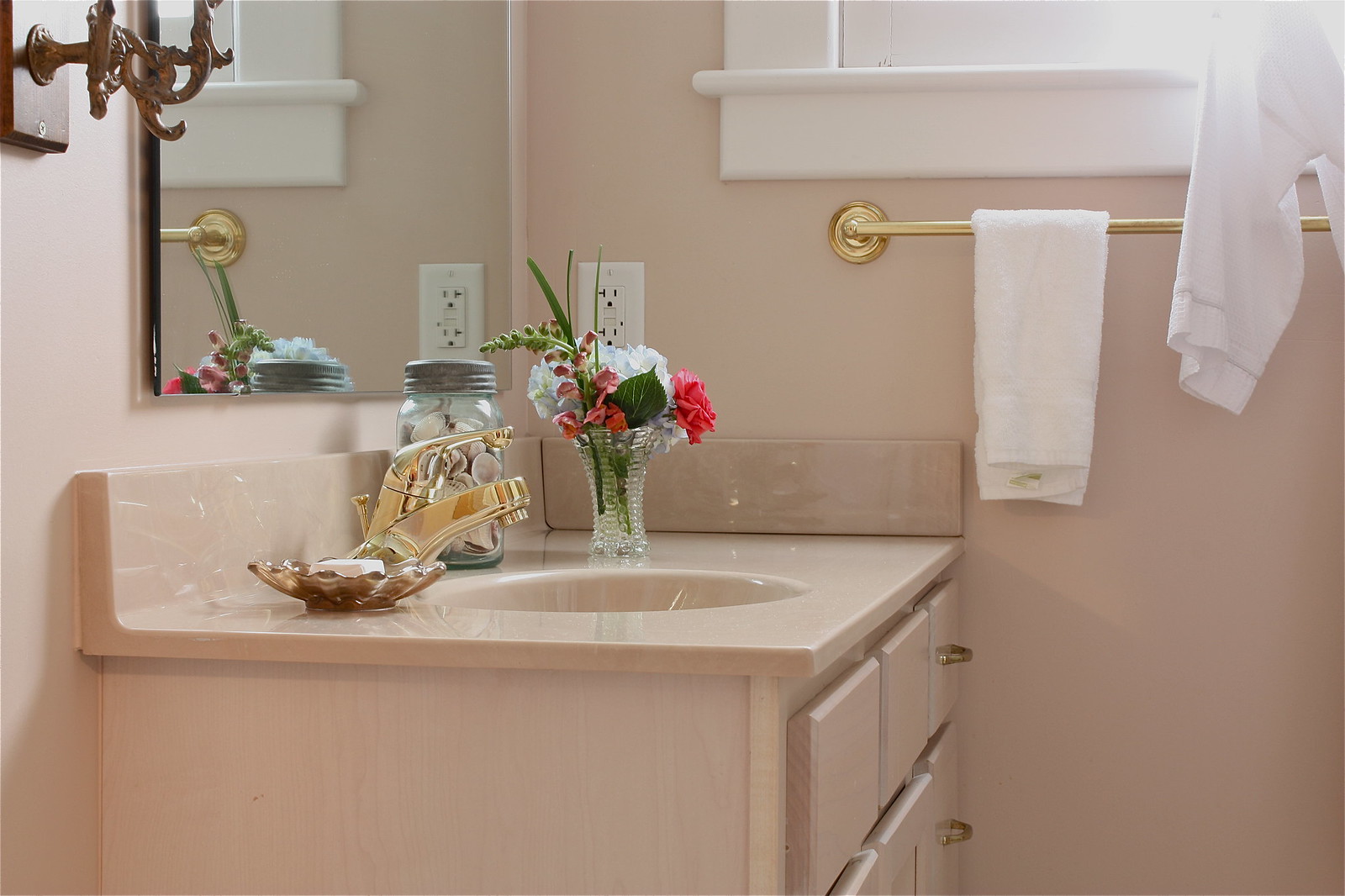A charming corner bathroom exudes a soft, delicate ambiance with its pale pink walls, countertop, and cabinets. The elegant vanity features a gold faucet paired with a clear vase filled with fresh white and pink flowers, adding a touch of natural beauty. A seashell dish to the left of the faucet holds soap, blending practicality with a coastal aesthetic. The cabinetry is adorned with gold hardware, harmonizing perfectly with the faucet's luxurious finish. Behind the sink, a mirror reflects the serene setup, while a white windowsill peeks out from above, holding a window whose frame isn't fully visible in the picture. Below the window hangs a neatly folded white towel on a gold towel rack. The photograph is cropped about a foot and a half past the right side of the sink, focusing on the neatly designed and intimate space.